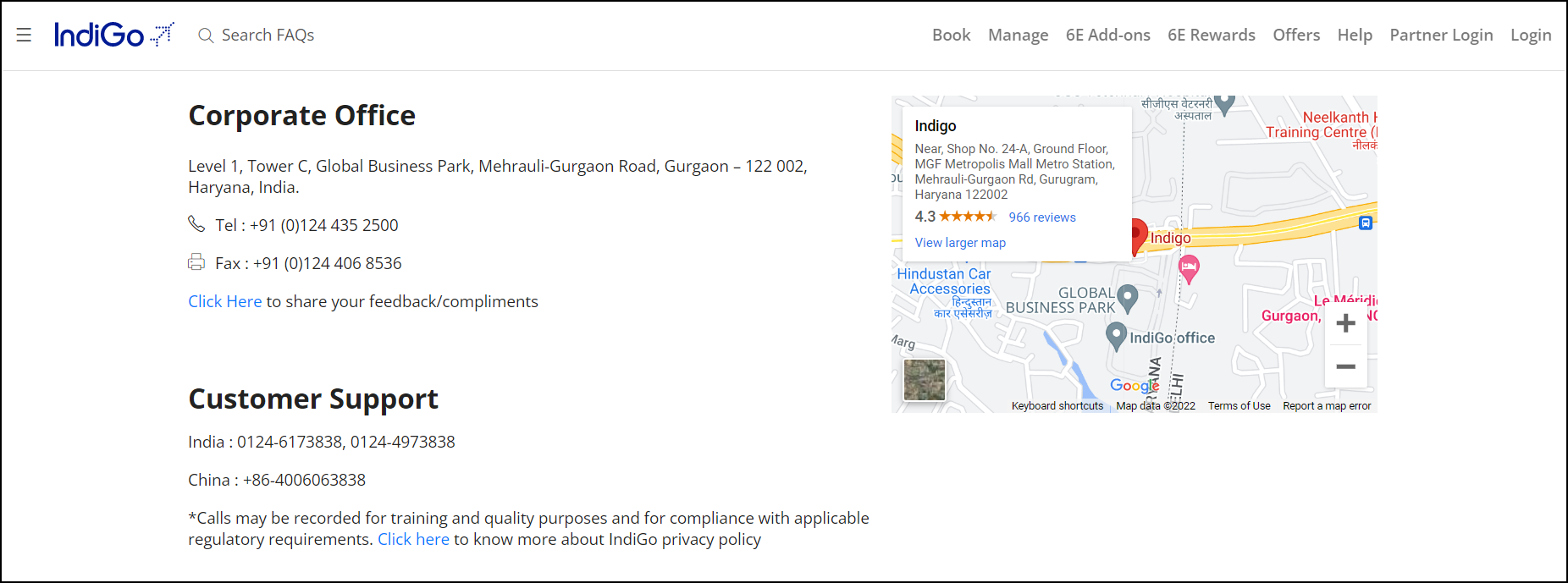Screenshot of the IndiGo Airline's corporate information webpage. The top section prominently displays the IndiGo logo, spelled "I-N-D-I" followed by a capital "G-O", accompanied by a small airplane icon, suggesting it is an airline company. In the upper right-hand corner, there are several navigation links including "Book", "Manage", "6E Add-ons", "6E Rewards", "Offers", "Help", "Partner Login", and "Log In".

On the left side of the page, a header labeled "Corporate Office" provides the location details: Haryana, India, accompanied by a telephone number and a fax number. There are also links for sharing feedback and compliments. Below this section, customer support numbers are listed for both India and China, with a note indicating that calls may be recorded for training and quality purposes. A blue hyperlink is available for users to learn more about IndiGo's privacy policy.

The right-hand portion of the screenshot features a Google Map highlighting the precise location of IndiGo's corporate office, alongside nearby points of interest. The webpage is dedicated solely to providing corporate contact information and customer support details, with the map enhancing the geographical context of IndiGo's headquarters.